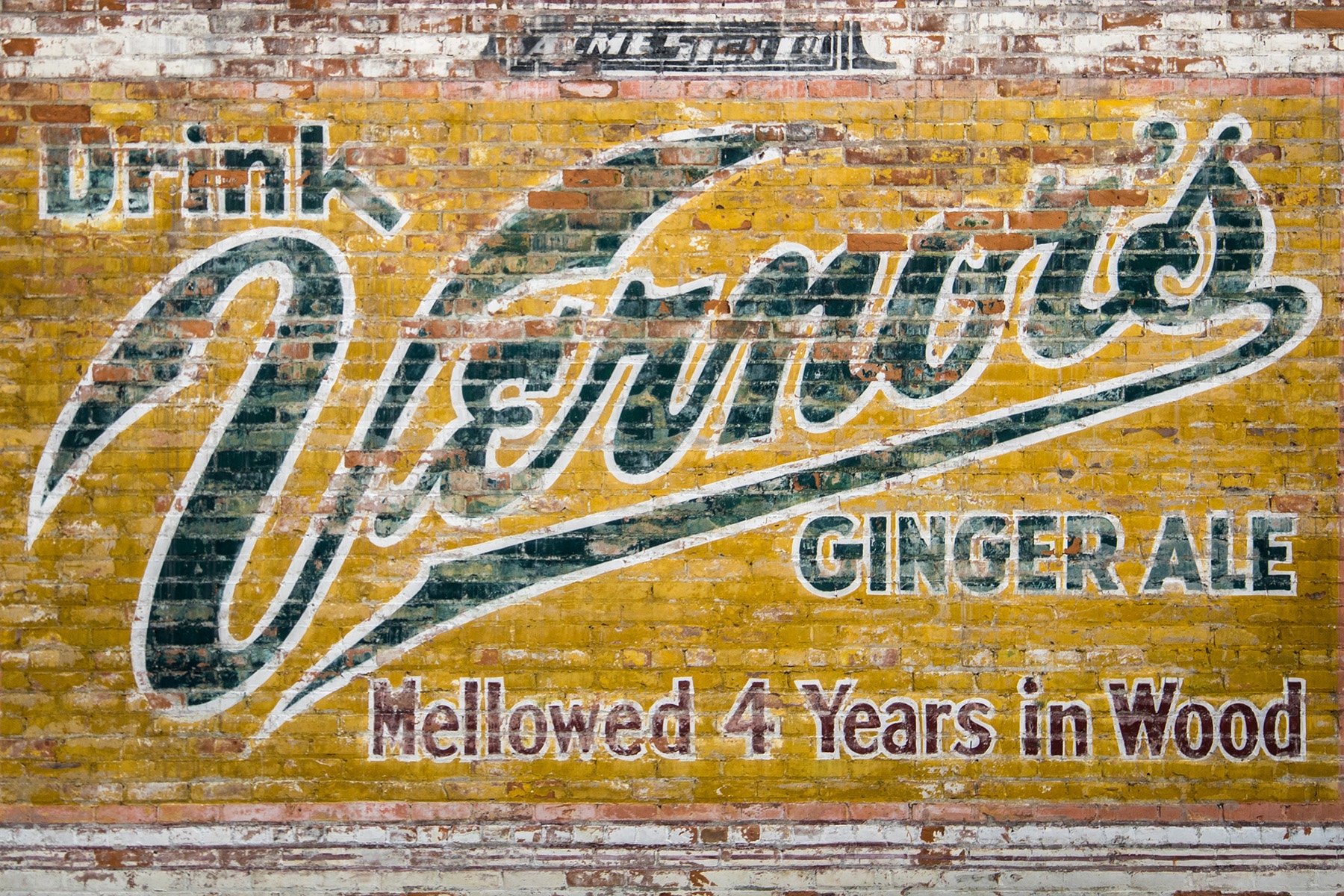This photograph captures a faded advertisement painted on an orange brick wall of a building, possibly located near an alley as there are no windows disrupting the surface. The advertisement features a large, worn yellow background that dominates the wall almost from top to bottom. At the top of this vintage mural, there is a black banner that likely once read "Acme Sign Co.," although it is now heavily faded and difficult to decipher. 

The main text of the advertisement is in green, cursive lettering and reads "Drink Vernors," with the letters "V-E-R-N-O-R-S" extending diagonally, and the tail of the "S" looping back towards the beginning of the word. Directly beneath this, in uppercase green letters with a white outline, it says "Ginger Ale." At the very bottom, in red text also outlined in white, the slogan "Mellowed Four Years in Wood" is prominently displayed. Despite its worn appearance, the advertisement's intricate design and nostalgic charm remain a captivating sight.